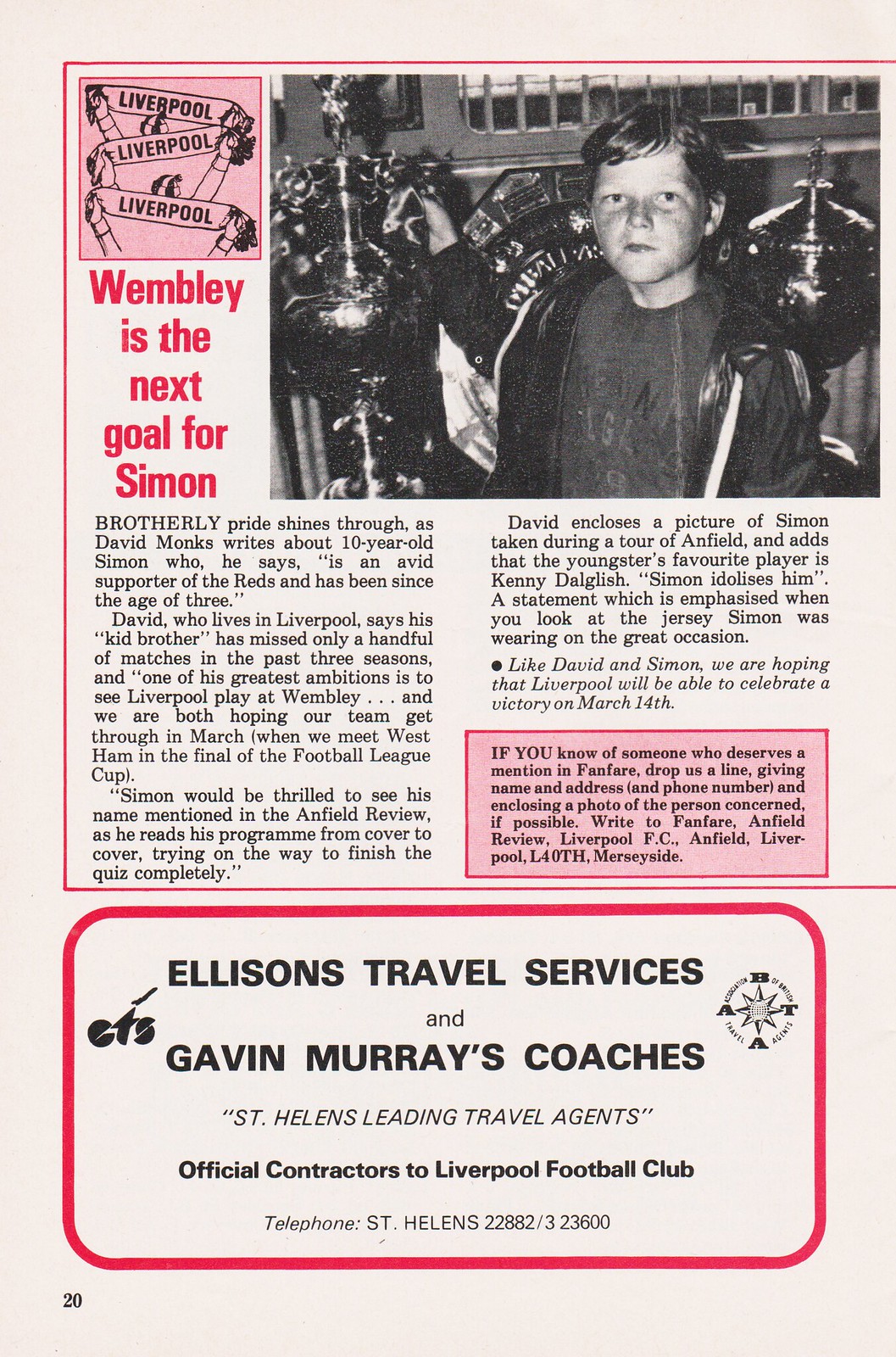The image depicts a page from a Liverpool Football Club program. On the left side, there is the Liverpool FC logo accompanied by the word "Liverpool" written three times, designed to resemble animated figures. The right side features a black-and-white photo of a young boy, identified as 10-year-old Simon, holding a sports trophy with additional trophies in the background. The title of the article reads "Wembley is the Next Goal for Simon," authored by David Monks. The article highlights Simon's deep commitment to the Reds, which began at the age of three. David narrates with brotherly pride about how Simon scarcely missed any major matches last season and expresses their shared aspiration to witness Liverpool play at Wembley, particularly emphasizing the upcoming Football League Cup final against West Ham. David also mentions Simon’s enthusiasm for reading the program cover to cover, attempting quizzes, and idolizing player Kenny Dalglish. The page also includes an advertisement for Ellison’s Travel Services and Gavin Murray's Coaches, noted as St. Helen's leading travel agents and official contractors to Liverpool FC, with a contact telephone number provided.